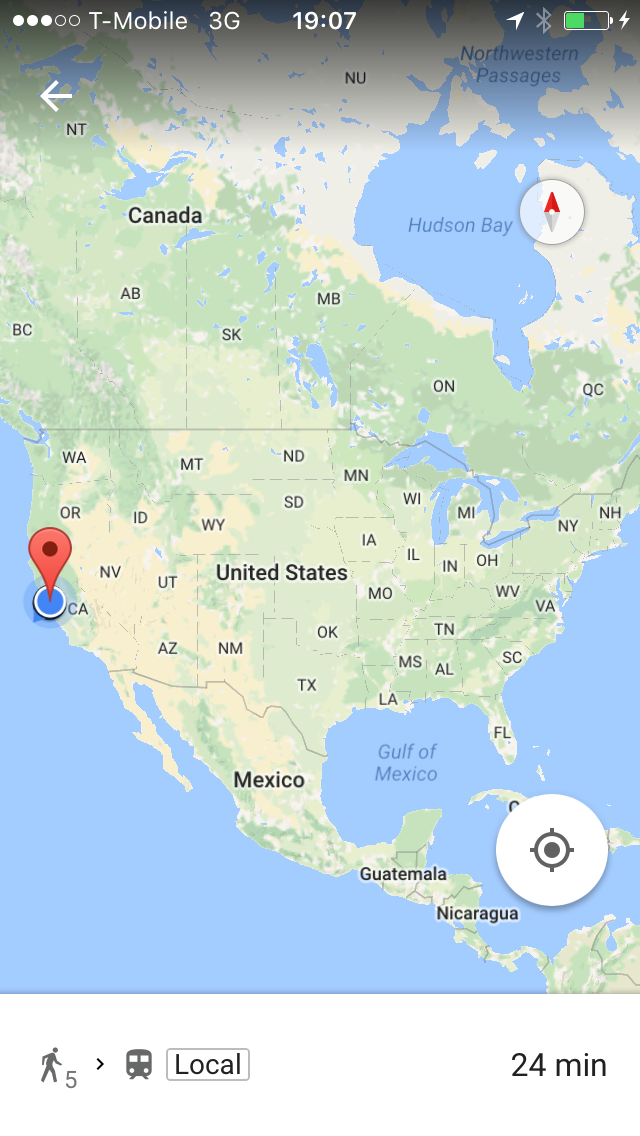The image is a detailed screenshot of Google Maps taken from a mobile phone. At the top left corner, there are three dots followed by two hollow dots. Next to that, it displays "T-Mobile" and "3G," the time "19:07," an arrow pointing upright, a blue symbol, a partially-filled green battery icon with a lightning symbol indicating charging on the right. The map itself shows the entirety of the United States, with Canada, Mexico, Guatemala, and Nicaragua labeled as well. A little red pin mark indicates a location in California. At the bottom, an icon of a person walking with the number "5" next to it and a bus labeled "local" show that the route includes walking and a bus ride, totaling 24 minutes. Additional map features include the Hudson Bay near Ontario and Quebec, and the northwestern passages. There is also a compass marker on the image.